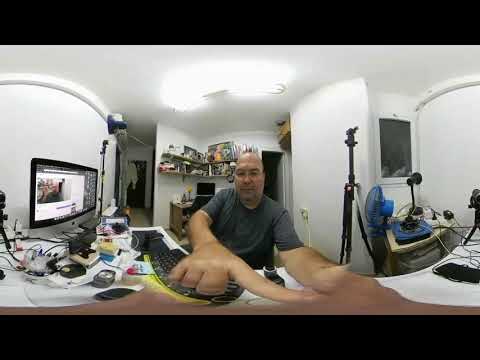In this panoramic indoor image of a home office, the scene is centered around a light-skinned, bald man wearing a gray t-shirt, who is seated at a desk in front of an Apple computer. His right hand extends towards the center of the image, creating a distorted effect characteristic of a 360-degree photo. The office appears cluttered, with various media and camera equipment scattered around. On the left side, the man’s desk is equipped with a black keyboard and a computer against a white wall. The desk surface is messy with numerous items on it. To the right, there's another desk with more photography gear, including several tripods and a blue fan, lending the area an impression of a small photography studio. Behind the man, positioned in the center background, is another desk topped with a computer and flanked by two shelves densely decorated with pictures and assorted items. Two doors are also visible in the back. The screen of the man's computer displays a YouTube video featuring himself, identifiable by the same background setup of artwork and shelving seen in the room.